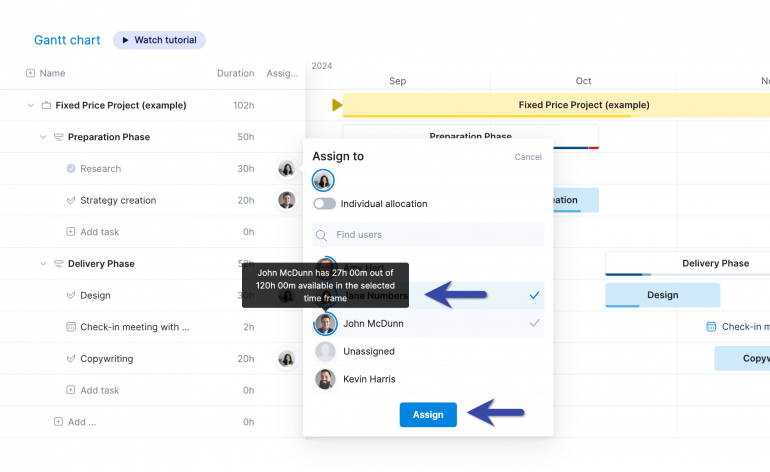The image depicts a comprehensive tutorial on creating a Gantt chart. In the upper left-hand corner of the screen, the words "Gantt Chart" are displayed prominently in a blue font. Adjacent to this, a gray oval-shaped rectangle contains the text "Watch Tutorial" in dark blue, accompanied by a small arrow icon indicative of a video play button.

The layout features two main columns: the left-hand column lists various elements that can be included in a Gantt chart, each with linked tutorials for further guidance. The right-hand column appears to show detailed instructions or visual aids related to the selected Gantt chart component.

Centrally, a pop-up box has appeared, highlighting functionality that allows for assigning different segments of the tutorial to various users. This specific instance shows another overlay message indicating that "John McDonne" has a particular section assigned to him. The overall image serves as an instructional guide, visually detailing how to navigate and utilize the Gantt chart tutorial effectively.